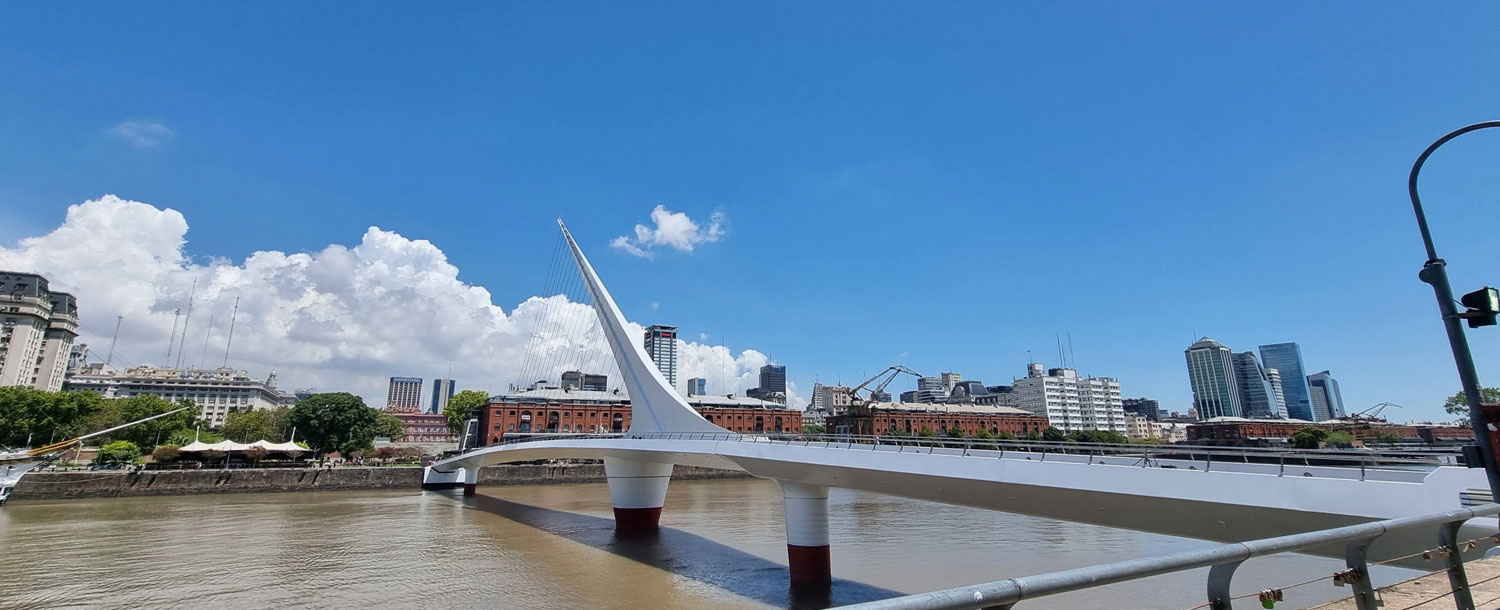This horizontal panoramic color photograph captures a walking bridge spanning a muddy brown river against a vibrant urban skyline. The bridge, seemingly designed for pedestrians and painted silver or white, features a prominent architectural element on top resembling the tail of an airplane or a spike. This structure extends into the sky and is supported by metal cables. The bridge surface has shadows cast by the bright sunlight, further highlighting its newly constructed appearance. On the horizon, a large, fluffy cumulonimbus cloud decorates a mostly blue sky. The cityscape across the river comprises a mix of buildings, some towering up to 20 stories while others are shorter, resembling old warehouses, adding historical texture to the scene. The photograph exhibits slight distortion, causing the buildings to appear somewhat skewed. A metal railing is visible on the bridge, and despite its inviting pathway, no pedestrians are present.